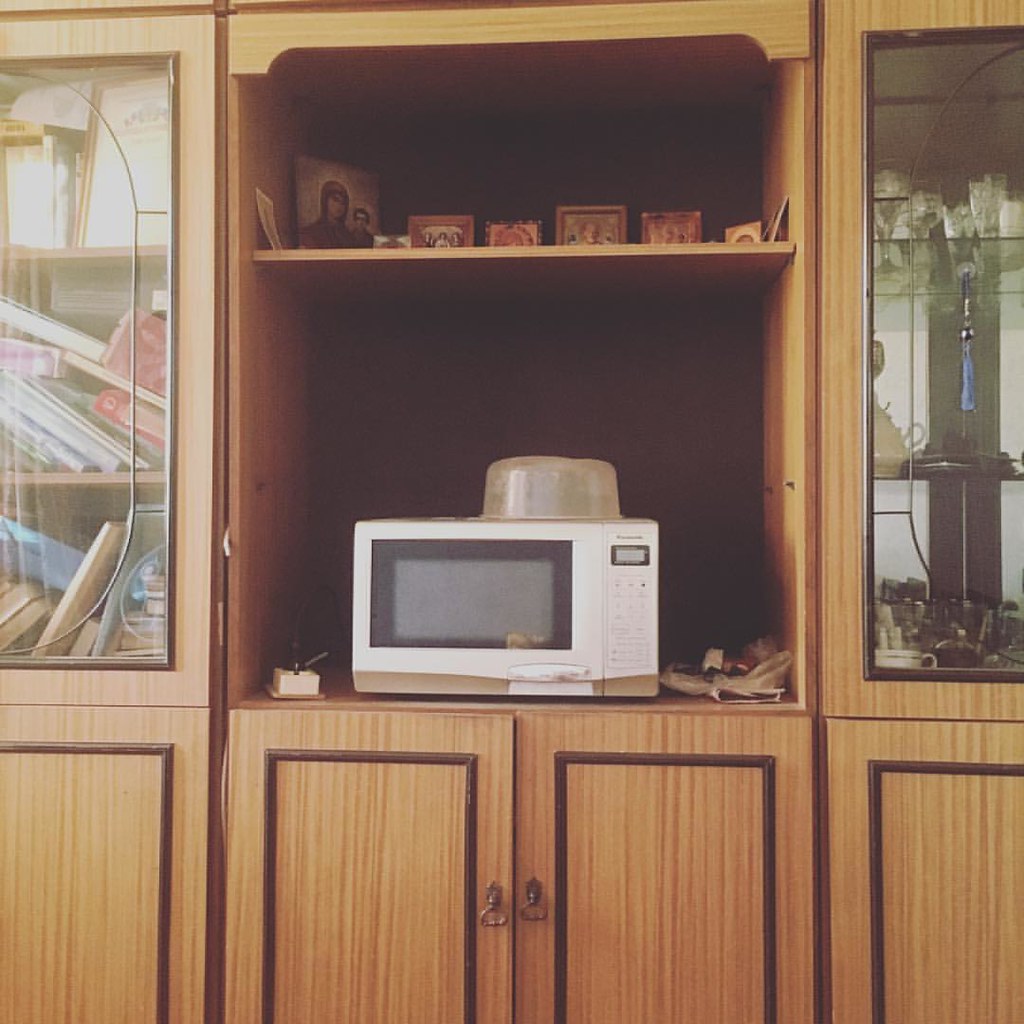In the center of the image is a white microwave with black trim, located on the lower shelf of an open cabinet space. On top of the microwave, there's an upside-down, see-through plastic container with a yellowish-orange tint. The microwave sits amid a larger brown cabinet unit that has bronze handles and black trim on its doors. Flanked on either side of the open space are glass-paned cabinets: the right one contains neatly arranged stemware and possibly other glass items, while the left one holds a messy, leaning stack of books and small boxes.

Above the microwave, the upper shelf is populated with various iconography and photos, primarily featuring religious or saintly figures, though some appear to be family members in smaller frames. Surrounding the central open portion of the cabinet, the lower part of the image shows two doors with dark outliner trim forming a rectangle, featuring door pulls at the center. The overall arrangement suggests a mixture of utility and personal memorabilia, blending kitchen or living room storage with an array of personal and decorative items.